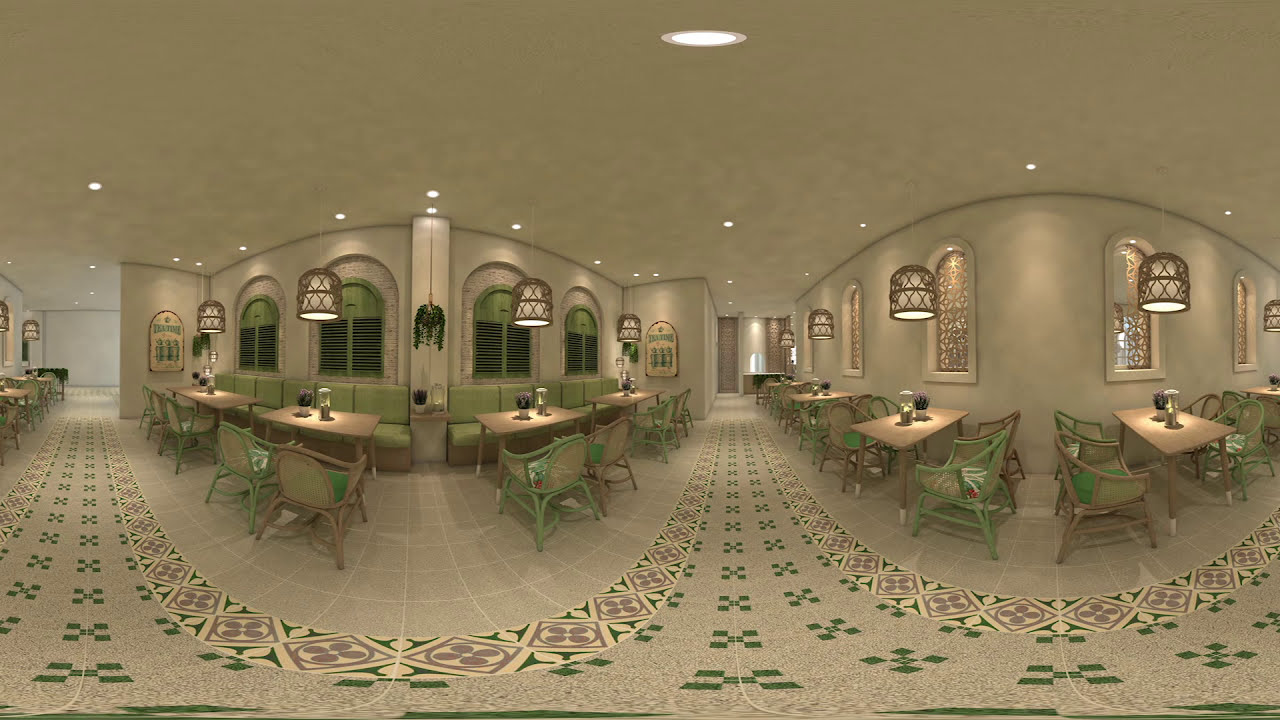The image depicts a panoramic, eggshell-colored cafe with a natural, earthy aesthetic. The floor features a beige and green tiled pattern with intricate designs, such as brown petals and four-leaf clovers. Lining both sides of the cafe are wooden tables with green and beige chairs or green sofas, each table illuminated by a domed hanging light. The walls, made of tan clay, are adorned with gold-arched windows featuring spiral designs and crisscross patterns. The ceiling mirrors the floor's light beige hue, with tiny white lights studded overhead. The seating includes curved booths on one side and additional tables against the far walls, all maintaining the light green and light brown color scheme. In the center back, an entrance doorway is visible, enhancing the symmetry and welcoming feel of the space.